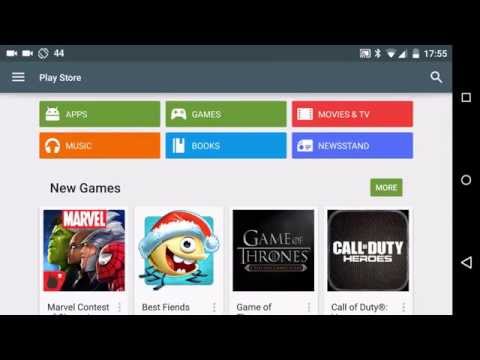This detailed image, captured on a mobile device held in a horizontal orientation (indicated by the device buttons situated on the right side), features the interface of the Google Play Store. At the top of the screen, the familiar "Play Store" label is prominently displayed, flanked by an unopened hamburger menu on its left and a search icon on its right. The main content of the screen is organized into two distinct rows of buttons. 

The first row displays three buttons labeled "Apps," "Games," and "Movies & TV" from left to right. Directly below, the second row features buttons labeled "Music," "Books," and "Newsstand." Beneath these rows, a "New Games" section is highlighted, with a "More" button positioned to its right. Within this section, the thumbnails of four different games are visible, each represented by a unique image, inviting users to explore new gaming options available on the Play Store.